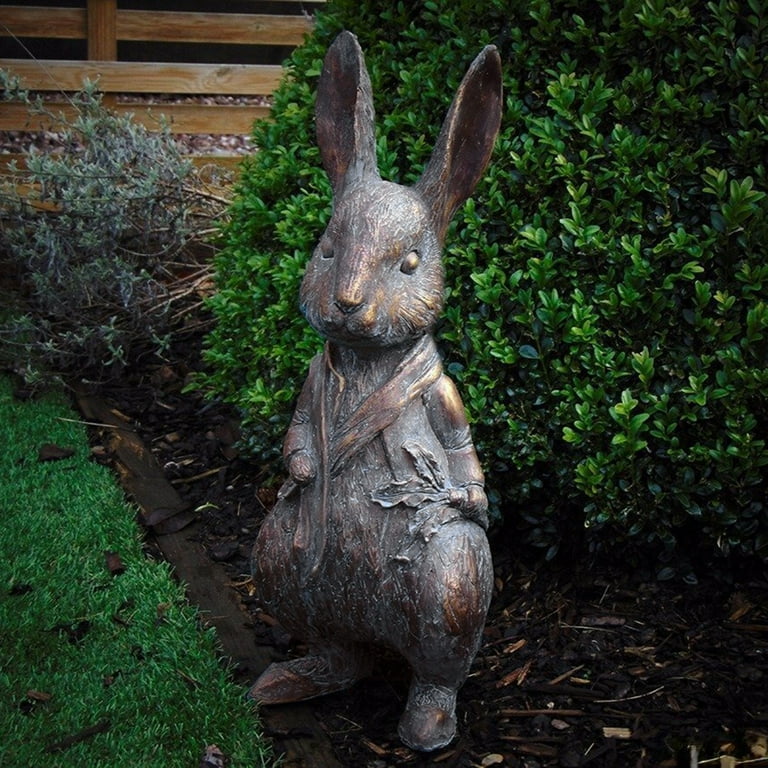This depiction showcases a bronze-toned statue of Peter Rabbit, standing approximately two feet tall, situated in a meticulously landscaped garden. The curious rabbit, his ears pointed straight up, gazes at the viewer with a subtly relaxed expression, his head slightly cocked. Peter is adorned in a jacket and scarf, with his left hand clutching a carrot – its leaves draped across his belly – and his right hand gently holding his scarf atop his vest. He stands on a neatly contained bed of brown mulch, bordered by a specifically designated landscaping area that separates it from lush, well-cut green grass. Adjacent to Peter, a neatly trimmed boxwood shrub and a slightly withered rosemary bush enhance the garden's aesthetic. The backdrop features a rustic, unpainted wooden fence, adding to the overall charm of the carefully maintained yard.